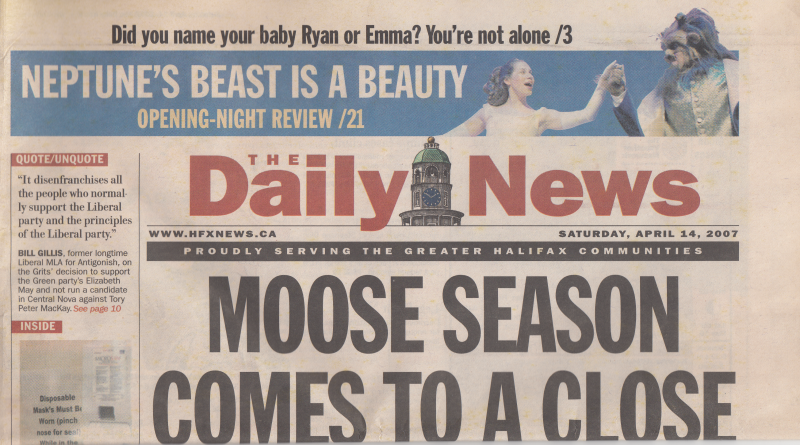**Caption:**

The image is a screenshot of a newspaper page, about twice as wide as it is tall, with a light brown tint typical of aged newsprint. At the top, in bold black text, it asks, "Did you name your baby Ryan or Emma? You're not alone /3." Below this, a blue banner with white text proclaims, "Neptune's Beast is a Beauty," with a subheading in yellow text that reads, "Opening Night Review /21." 

To the right of the blue banner, there is a photograph of two actors, presumably from the play mentioned, with one actor holding the other's hand, both seemingly in the midst of a song. Centered beneath this image, vivid red text spells out "The Daily News," flanked by a clock tower emblem between "Daily" and "News". 

An all-black banner beneath this central section states, "Serving the Greater Halifax Communities." Dominating the bottom portion of the page, about 40%, two prominent lines of text in large black capital letters announce, "MOOSE SEASON" on one line and "COMES TO A CLOSE" on the next line.

The upper left corner of the page lists a website, while the upper right corner notes the date: "Saturday, April 14th, 2007." Down the left margin, beneath a section labeled "Quotes" and "Inside," are a couple of blurbs, details of which are unspecified.